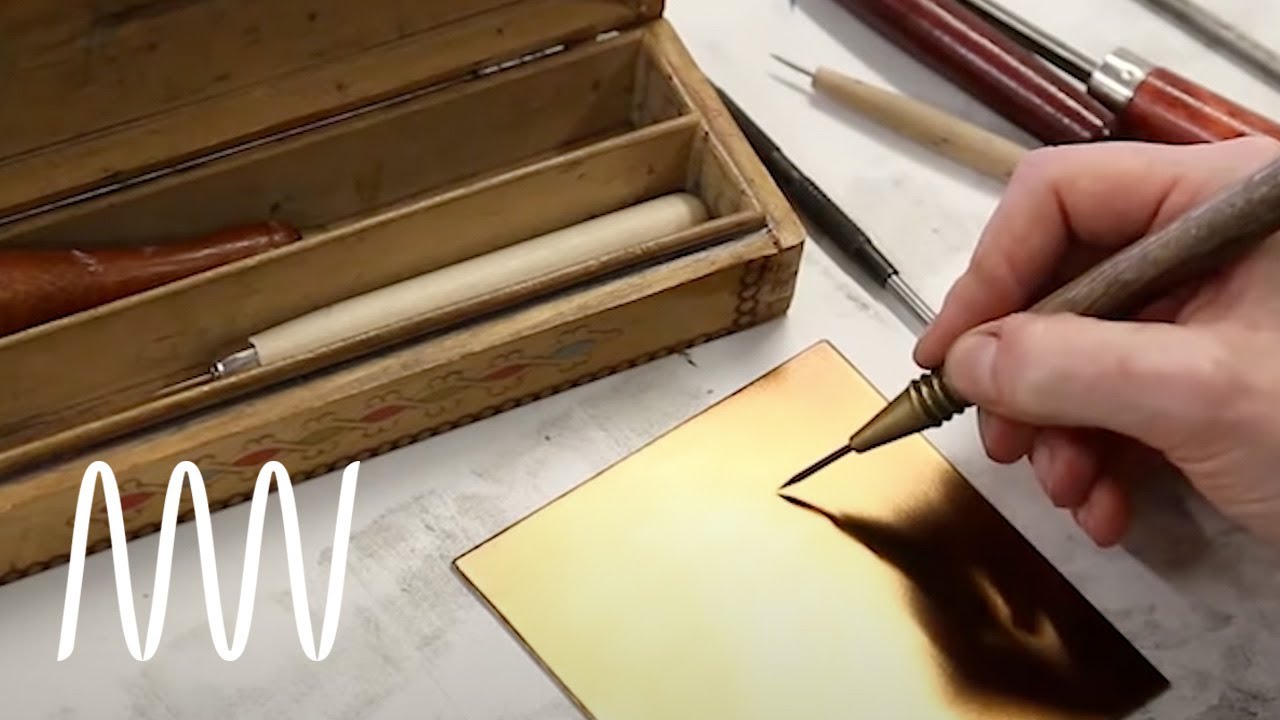In this image, an artist is depicted beginning the intricate process of hand engraving or etching on a gold-colored metal plate, likely brass, placed atop a wooden table. The artist's right hand grips a specialized etching tool, characterized by a sharp metal tip emerging from a metal cone base attached to a wooden handle, poised delicately near the plate's surface. Surrounding the central image are various additional tools, each with unique wooden handles in shades ranging from off-white to deep mahogany and reddish brown. To the side, there’s a wooden storage box with compartments containing more etching tools, emphasizing the craft's detail-oriented nature. In the bottom left corner, a white logo resembling an intertwined cursive M and W stands out against the background, suggesting a possible branding or advertisement context. The entire scene is set on a neat, white and grayish countertop that contrasts subtly with the wooden and metallic elements of the engraving setup.